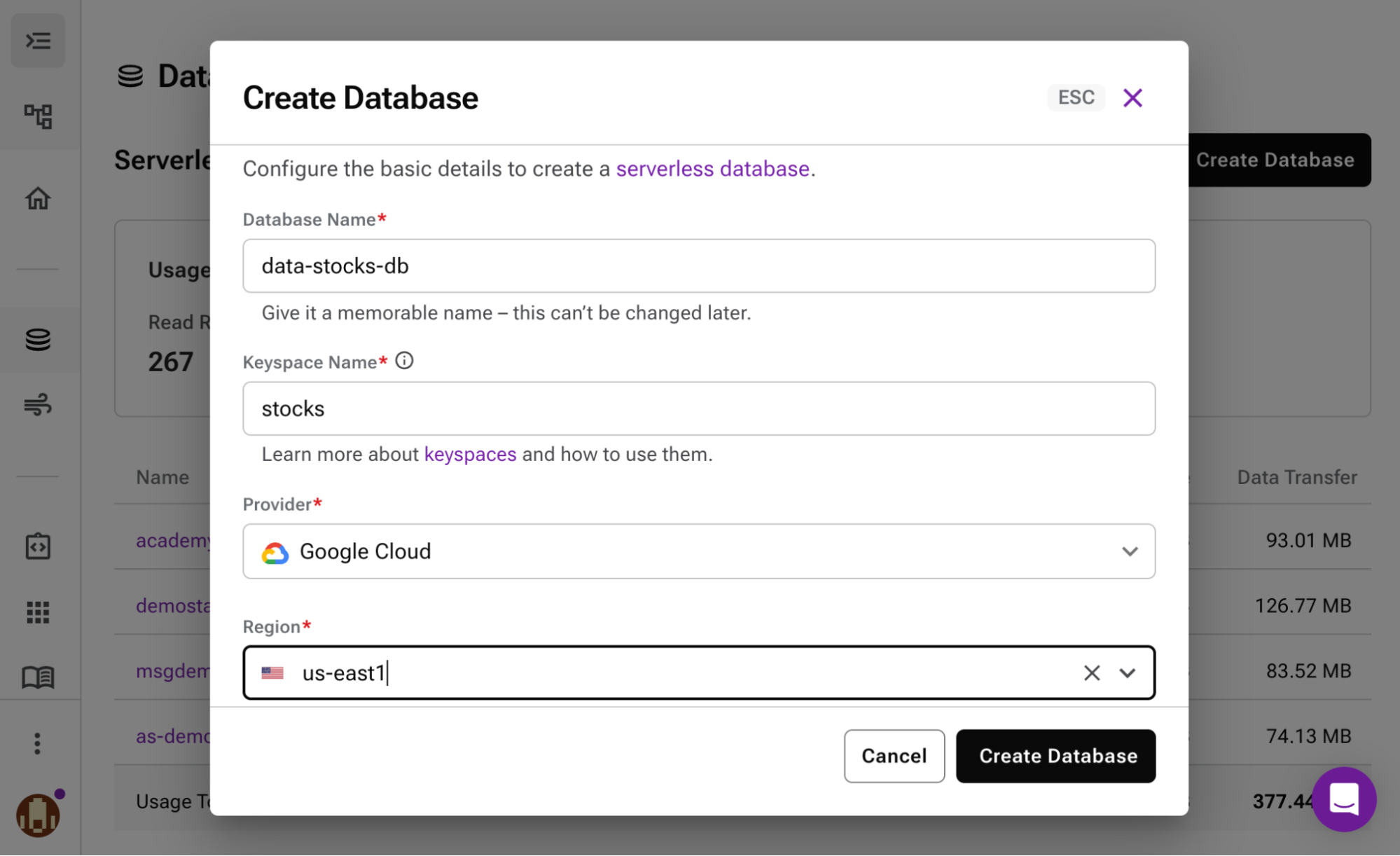This is a screenshot of a website interface where a popup window titled "Create Database" is displayed in black text. Beneath the title, in smaller text, it explains: "Configure the basic details to create a serverless database," with the phrase "serverless database" highlighted in purple. 

The first field is "Database Name," marked by a red asterisk indicating it is required. The chosen name for the database is "datastocksdb." Below this field, a note mentions, "Give it a memorable name; this can't be changed later on."

The next field is "Keyspace Name," also required and marked by a red asterisk. The entered keyspace name is "stocks," accompanied by a prompt in purple text that reads "Learn more about keyspaces and how to use them."

Following this, the "Provider" field, which is also mandatory, shows that "Google Cloud" has been selected. It appears to be a drop-down menu from which different providers can be chosen. 

The last field is "Region," additionally marked with a red asterisk, indicating that "US East 1" has been selected.

At the bottom of the popup are two buttons: "Create Database" and "Cancel," offering the final actions for the user.